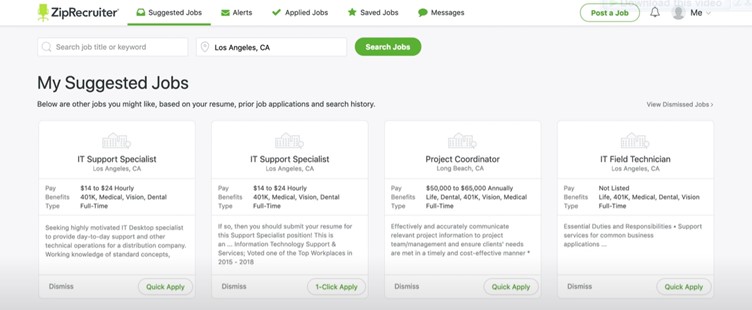The image displays a web page from Zip Recruiter. At the top, there is a navigation bar featuring a logo on the top left, which consists of black text reading "Zip Recruiter" alongside a green silhouette of an office chair. Adjacent to the logo are navigation buttons, characterized by black text with icons to the left side. There are five categorized buttons in total, with the far-left button currently selected. On the top right of the navigation bar, there is a "Post a Job" button accompanied by a few icons, including an empty profile photo icon.

Below the navigation bar, there are two search fields: one for job titles and another for locations, followed by a "Search Jobs" button to the right. Underneath these search fields is a header reading "My Suggested Jobs." Beneath this header, there are four sections that provide job information, each on a white background. Each job section lists the job title at the top center, followed by the location below it, and additional job details further down. At the bottom of each job section are two buttons for further actions.